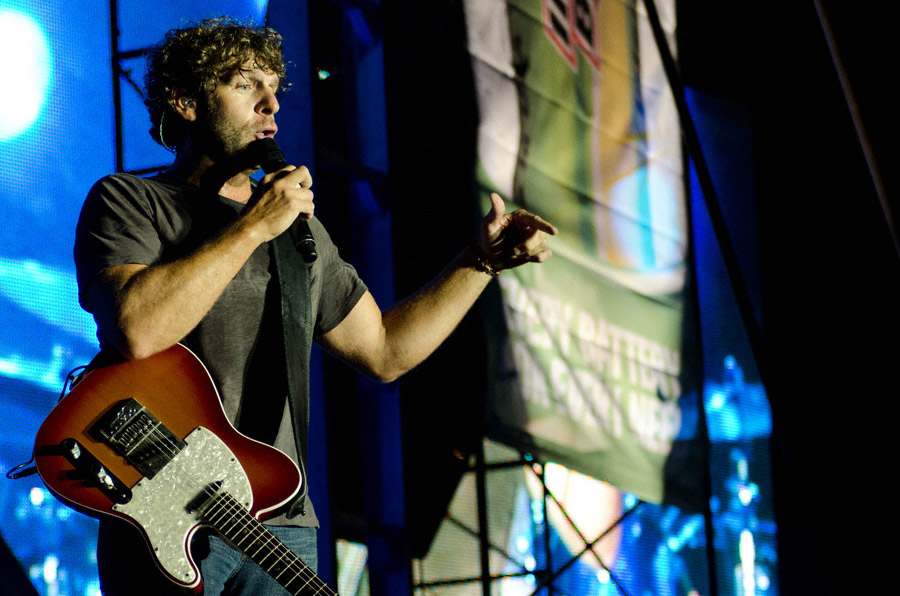The image captures a male musician on stage, positioned slightly left of center, engaging with the audience through a microphone held in his right hand. His left arm is raised, elbow bent at a 90-degree angle, with his thumb and fingers extended, gesturing towards the crowd. He has short, curly brown hair, a bit of beard and mustache, and is wearing a gray shirt. Draped over his shoulder by a black strap is an electric guitar featuring a black neck, brown body, and white accents with metal pickups, which rests against his side, pointing downwards. Behind him, multiple blue spotlights illuminate the stage, casting a vibrant blue hue across the background. A prominent banner hangs above, predominantly green and yellow, resembling a Bud Light Lime advertisement, with difficult-to-read white lettering across its various colored segments.